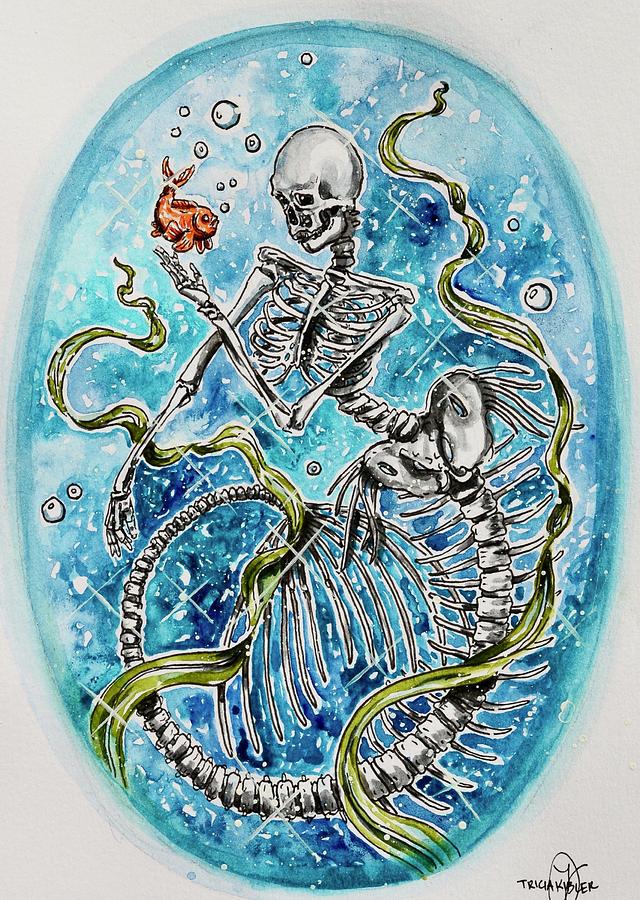This detailed hand-painted artwork by Tricia Kibler is framed within a blue oval, representing an underwater scene. The focal point is a white and gray mermaid skeleton with a spiraled tail, reaching out towards a small, vibrant goldfish that is facing it. The mermaid's skeletal arm extends under the fish, while the other arm hangs down. The scene is teeming with bubbles and pieces of seaweed, enhancing the underwater atmosphere. The fish and seaweed introduce splashes of color to the predominantly monochromatic skeleton, emphasizing the contrast. The artist's signature, "Tricia Kippler," is located at the bottom right corner, confirming the piece’s authenticity.